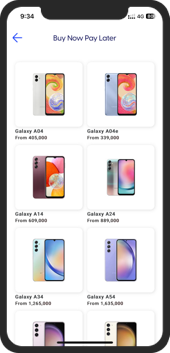The screenshot displays a smartphone screen with the current time of 9:34 and a partially obscured battery life indicator, suggesting a low charge. The interface, primarily white, showcases a list of Samsung Galaxy phones available for purchase. A blue arrow on the left offers a back-navigation option, while a blue-gray button indicates a "buy now, pay later" scheme.

Beneath this navigation bar, several models of Galaxy phones are presented, each adorned with a distinct swirl pattern on their screens. The topmost listing features a Galaxy AG4, starting at a price point that appears to be ₦35,000, indicating a currency other than dollars. The next is a Galaxy AG4E, followed by various models like the Galaxy A14 listed at what seems to be ₦69,000, and a Galaxy A24 with a price that is either ₦20,000 or ₦89,000—difficult to decipher due to blurriness.

Each row continues with different Galaxy models, although the text remains somewhat fuzzy, suggesting a lower quality image. The caption humorously notes the irony if the image was taken with a Galaxy camera. Ultimately, the selection is entirely composed of Galaxy smartphones.